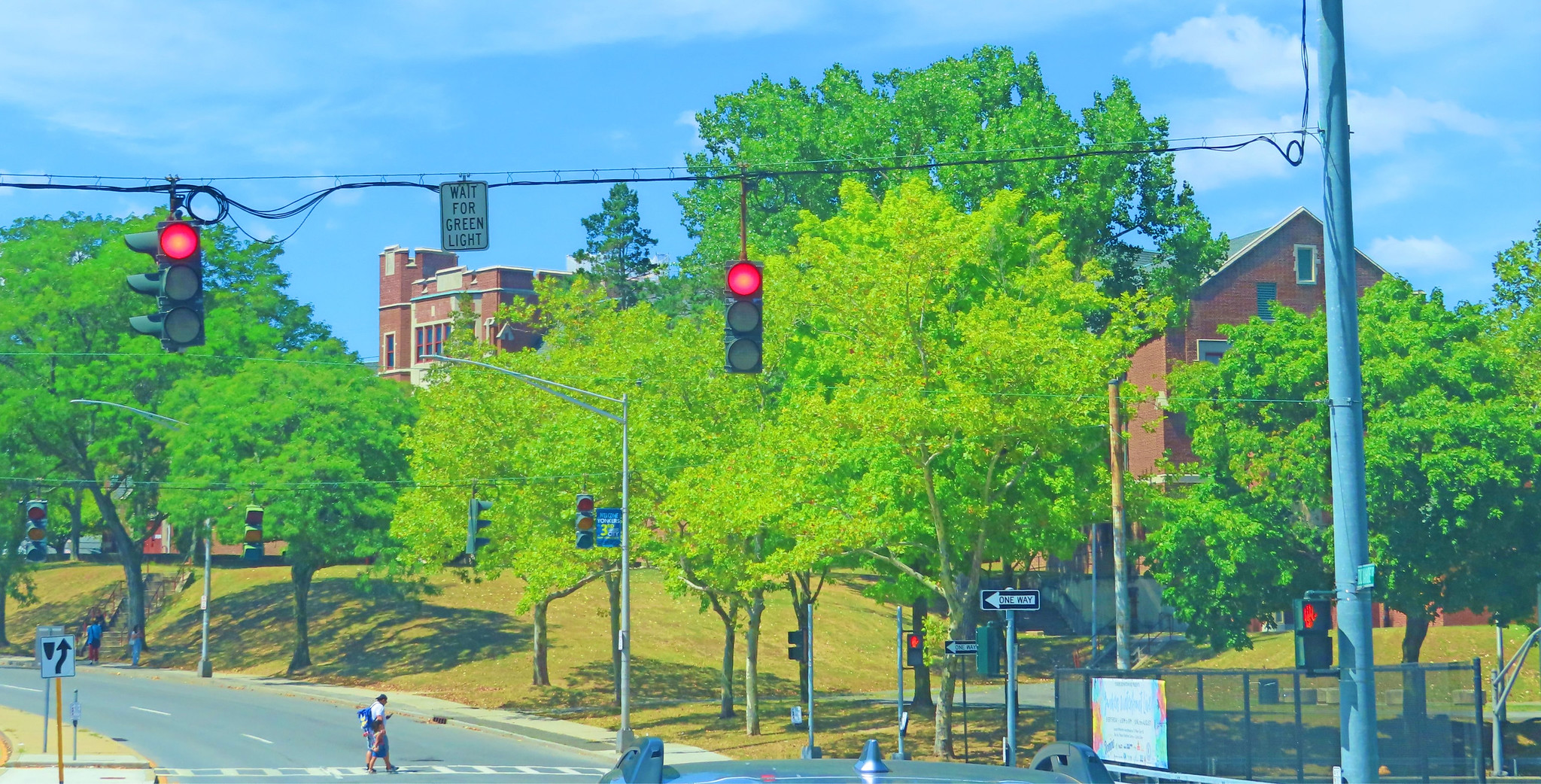The image captures a vibrant outdoor scene bathed in sunlight with a brilliant light blue sky accented by a few scattered clouds. In the upper half, two red traffic lights hang, connected by a wire, and a white sign in between them instructs, "Wait for green light." On the right side, a long blue-gray pole is visible with a "Do Not Walk" sign attached to it. 

The midsection showcases a rich collection of deciduous trees stretching horizontally across the image with splashes of green, and two brick buildings peek out from behind the foliage. One building, situated centrally, has a distinctive tower-like structure, while another, more burgundy in color, appears on the right side, resembling a farm building or campus structure.

In the foreground at the bottom, a two-lane road is present, and a person dressed in a white shirt, blue shorts, and a blue backpack is crossing the street. Another figure can be seen walking along the sidewalk, seemingly looking at their phone. The vivid colors of the trees and structures in the background add a striking contrast to the overall composition.